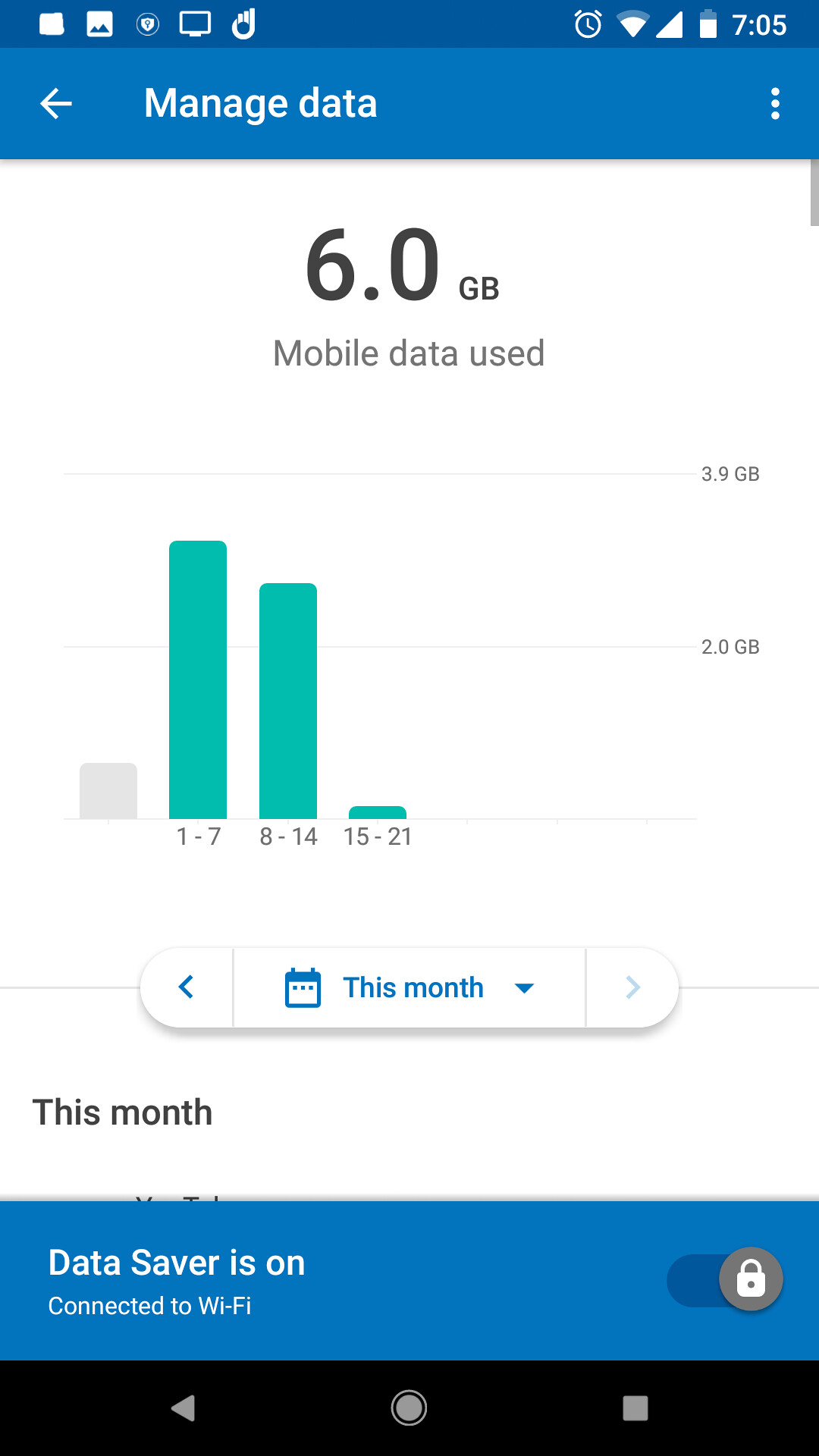This portrait-format, color screenshot displays a smartphone's "Managed Data" option within the control panel. The image reveals detailed information on mobile data usage, indicating a total consumption of 6.0 gigabytes. Usage is distributed across different periods of the month: the majority was used between the 1st and 7th, followed by a significant amount from the 8th to the 14th, and minimal usage from the 15th to the 21st, suggesting the data quota was reached by then.

The screen shows "Data Saver" mode as activated. The status bar at the top indicates the time is 7:05, and the device is connected to a Wi-Fi network. The visual elements of the screenshot include a predominantly white background, with key sections such as the "Managed Data" header and "Data Saver" status displayed in blue for emphasis.